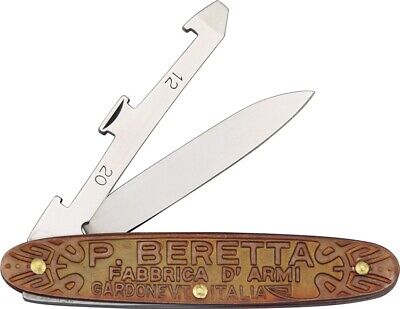The detailed close-up photograph captures a multi-purpose folding knife, prominently showcasing its craftsmanship. The knife's handle is a distinguished brown, possibly leather, adorned with intricate line patterns along its edges and secured by three gold studs, which hold the ensemble together. The handle bears an elaborate engraving that reads "P. Beretta Fabrica d'Armi," followed by "Gardone V.T., Italia." Partially extended from the handle are two silver blades: one a sharp knife blade, the other an intriguing tool engraved with the numbers 12 and 20, suggesting it serves a specific measuring purpose. Each element of the knife's design emphasizes both practicality and elegance, merging utility with refined Italian engineering.